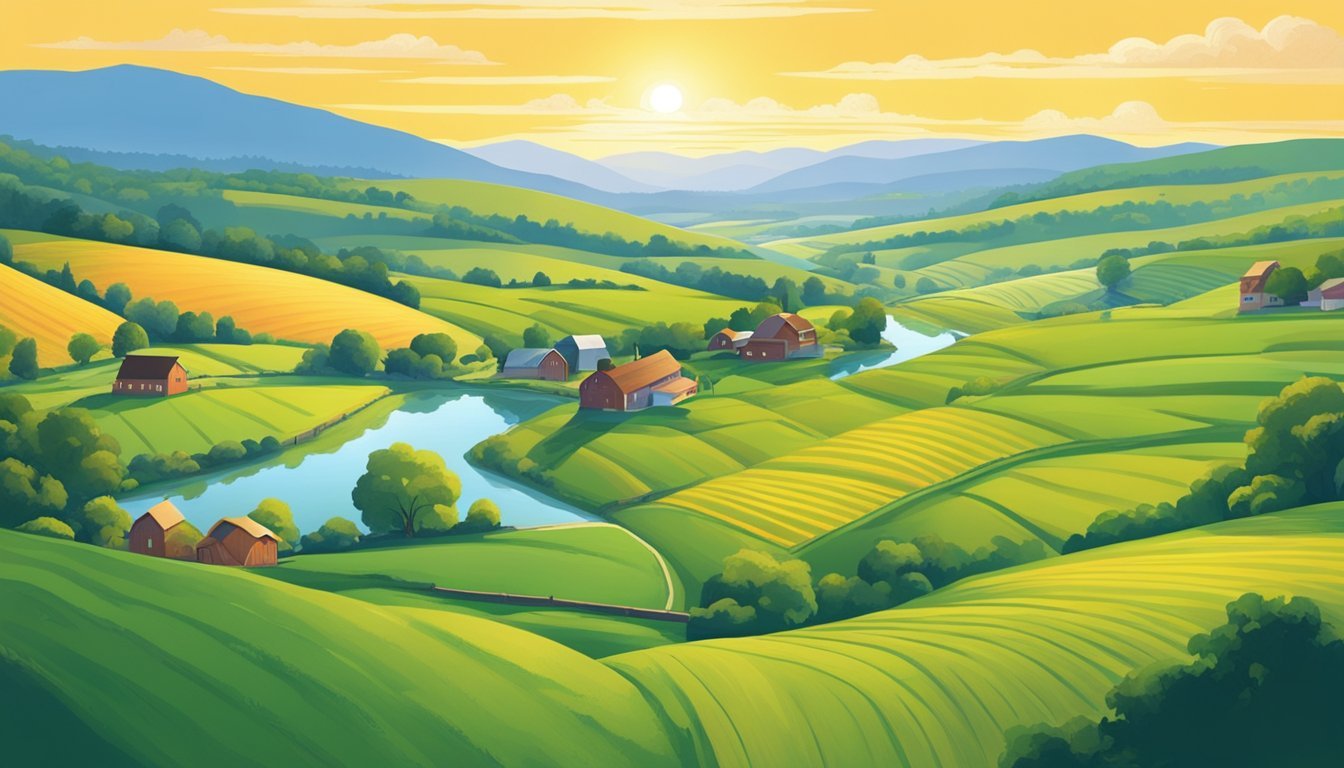The artwork presents a vibrant, idyllic landscape that appears to be a detailed painting or drawing. The sky is depicted in shades of yellow with wisps of white clouds, suggesting the aura of a setting sun, with a bright white sun positioned in the middle of the sky. Dark blue and gray mountains form a majestic backdrop, enhancing the composition's depth. In the foreground, rolling hills are painted in vivid green, accentuated with clusters of trees that give the scene a lush, fertile appearance. 

Centrally, a picturesque farm is illustrated with buildings in warm brown and red hues, including a house, barns, and a distinctive silver structure. A serene body of water meanders through the farm, linking to a sizable pond on the left, which is surrounded by more brown buildings and trees. To the right, another farm emerges, marked by similar rolling, green hills outlined with trees, further reinforcing the landscape's agricultural nature. Various farms and green pastures extend across the view, interconnected by the winding waterbody, creating a harmonious and visually appealing farmstead scene.